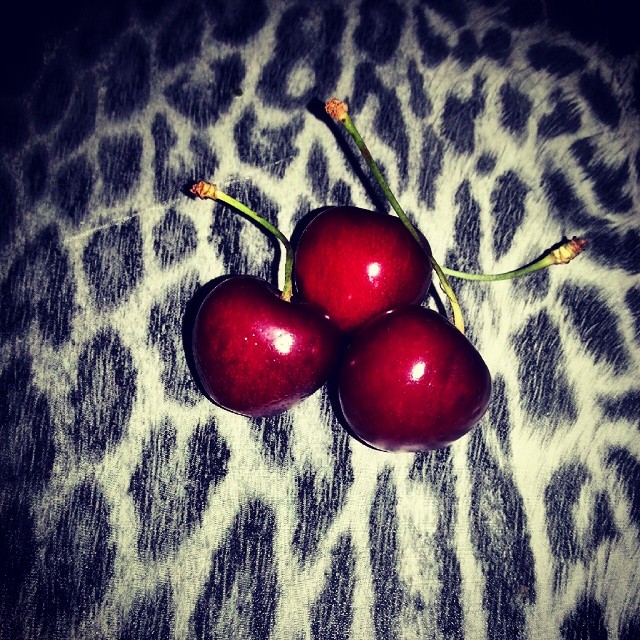This vibrant color photograph is an extreme close-up of three Bing cherries, arranged in a triangular formation with one on top and two at the bottom. The cherries, dark red with maroon hues that verge on black, have smooth, shiny surfaces punctuated by white dots reflecting the light above. Their thin, light green stems, which darken towards the center and tip with brown, suggest they've been freshly picked. The cherries are nestled close together on a white furry blanket that features irregular, navy blue, leopard-like spots. The detailed background not only adds texture to the composition but also emphasizes the lustrous and unblemished appearance of the cherries as they dominate the frame. The edges of the photograph are dark, drawing attention to the vividness and perfection of the cherries in the center.